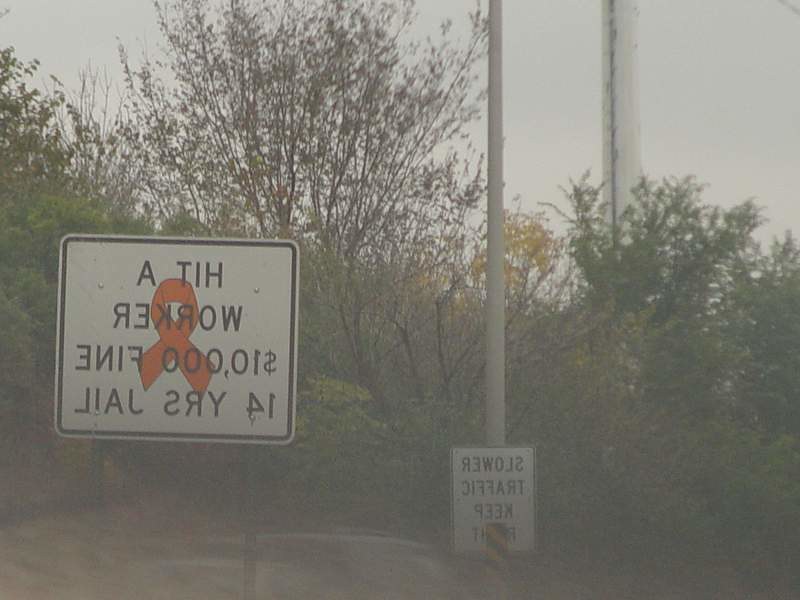This photograph captures an intriguing scene featuring two prominently displayed road signs. The first sign stands out with its white background and black text, adorned with an orange ribbon draped across it. Curiously, the text on this sign is inverted, adding an element of mystery. Adjacent to it, mounted on a white pole, is another sign also characterized by a white background and black text, with the text similarly reversed. In front of this pole-mounted sign, a small yellow sign with black stripes adds a splash of contrast.

The background of the image is dominated by a grove of trees, their lush green foliage interspersed with a starkly bare tree, devoid of leaves. Further in the distance, another tree displays leaves tinged with orange hues, hinting at an autumnal transition. The entire scene is enveloped in a muted, cloudy atmosphere, giving the photograph a washed-out, almost vintage appearance with colors that appear dull and slightly faded.